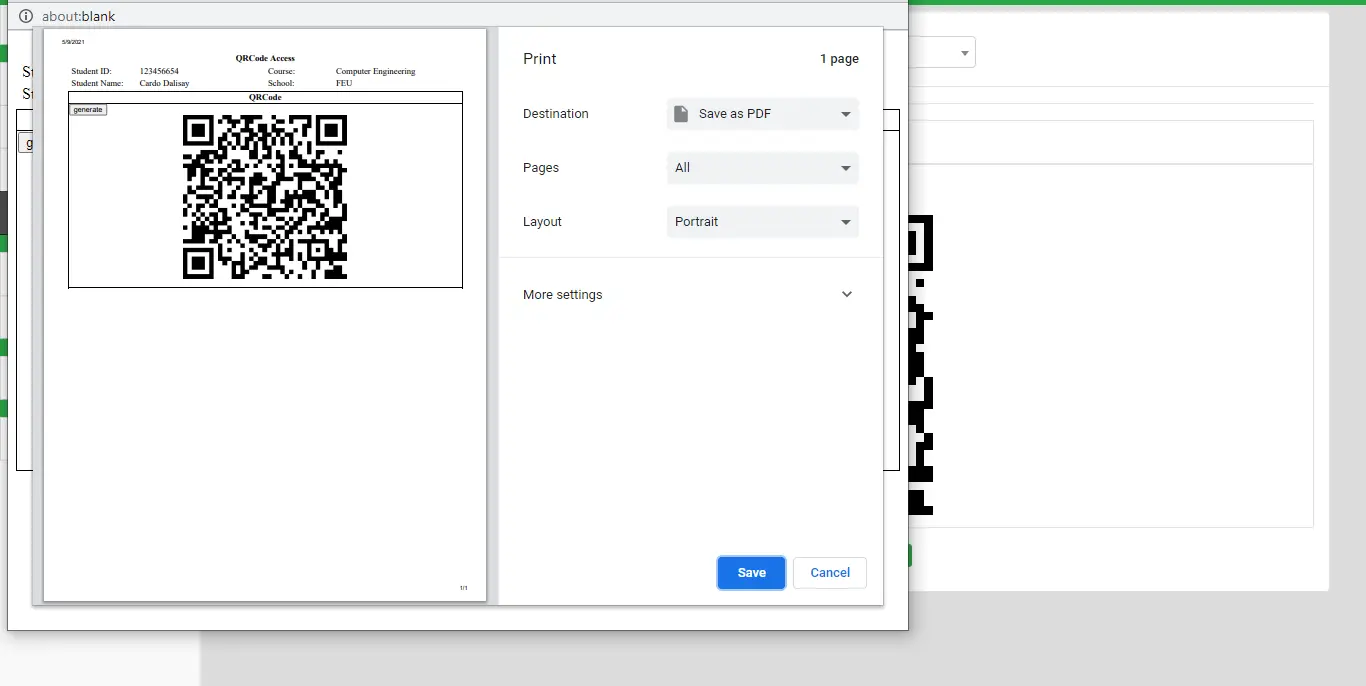This image displays a computer screen featuring a print dialog window. The main area is a horizontally oriented rectangle with a gray background. Dominating the center is a large white rectangle set against a black backdrop, containing portions of a QR code on the right side. Adjacent to this, another rectangular bubble with a light gray top extends out, displaying a similar QR code on its left side.

In the upper left corner of this dialog, the text "about:blank" is visible. To the right, the interface contains several print settings, including fields labeled "Print," "1 Page," "Destination: Save as PDF," "Pages: All," "Layout: Portrait," and "More settings."

At the bottom of the window, there are two clickable buttons. The first is a blue rectangle with the word "Save" written in white letters. The second button is outlined in a light gray (or possibly black) and is white, featuring the word "Cancel" in blue letters.